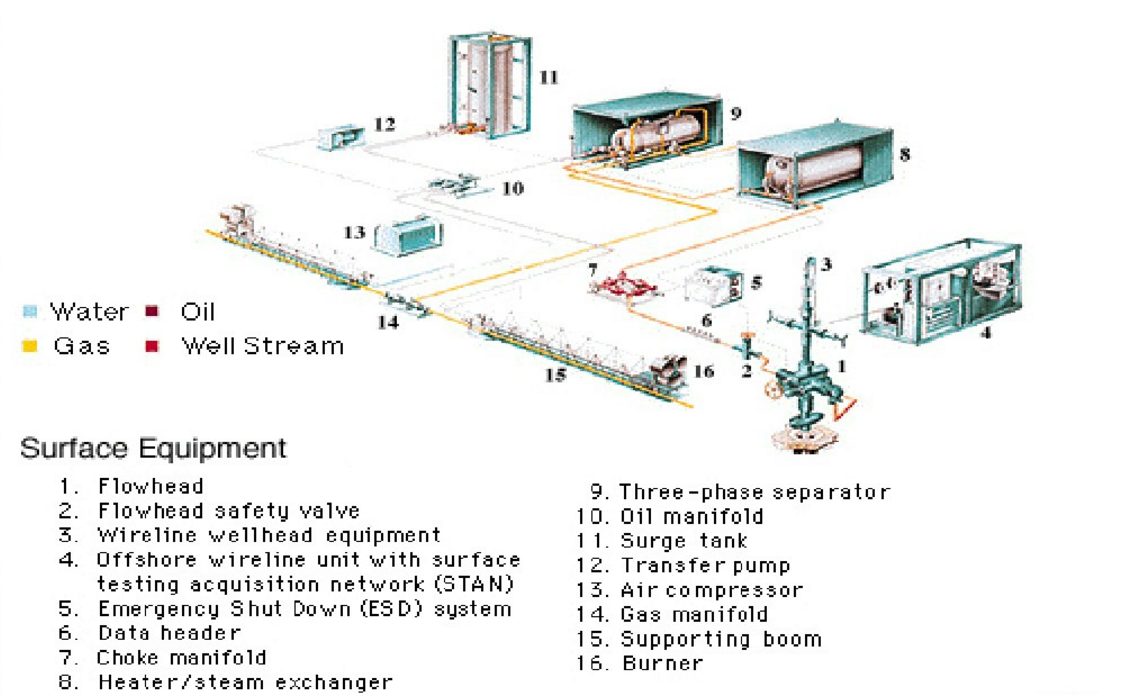The image is a detailed sketch of various components of machinery, specifically surface equipment used in the oil and gas industry. The sketch is mostly gray but includes color-coded elements to denote different substances: light blue for water, maroon for oil, yellow for gas, and red for the well stream. This color-coded system helps to identify the flow and type of each component within the machinery. 

The sketch is labeled with a title that reads "Surface Equipment" and includes a list of 16 items, each marked with a number and technical terms in a darker gray font, with the numbers in black. The equipment listed includes: 

1. Flow Head
2. Flow Head Safety Valve
3. Wire Line Well Head Equipment
4. Offshore Wire Line Unit with Surface Testing Acquisition Network (STAN)
5. Emergency Shutdown (ESD) System
6. Data Header
7. Choke Manifold
8. Heater or Steam Exchanger
9. Three-Phase Separator
10. Oil Manifold
11. Surge Tank
12. Transfer Pump
13. Air Compressor
14. Gas Manifold
15. Supporting Boom
16. Burner

The arrangement and detailed annotations give the impression of a well-organized work yard or industrial setup, highlighting the complexity and technical nature of these surface equipment components.